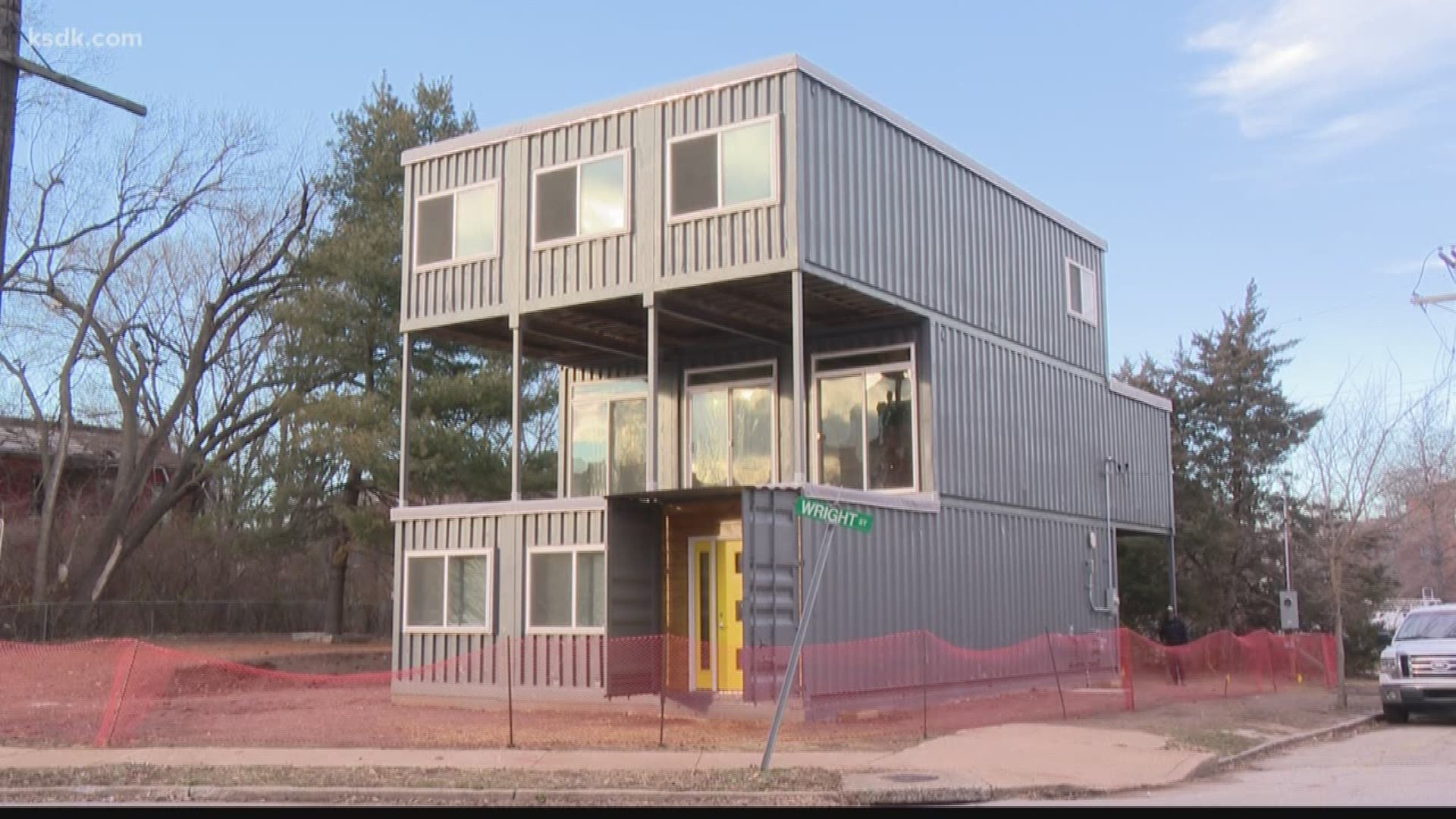This vertical rectangular image captures a highly unique modular home, appearing to be constructed from nine stacked shipping containers, all in a light gunmetal gray color. The residence is three stories high. The bottom level features a bright yellow door accompanied by two windows. The middle level is recessed, creating a balcony space with three large sliding glass doors, while the top level aligns with the bottom and is adorned with three horizontal windows. The entire structure is enclosed by an orange mesh construction fence, indicative of ongoing work. Situated on a dusty lot in Old North St. Louis, Missouri, the scene includes a green street sign for Wright Street, which is notably slanted. This innovative design exemplifies modern living through its distinct use of shipping containers.